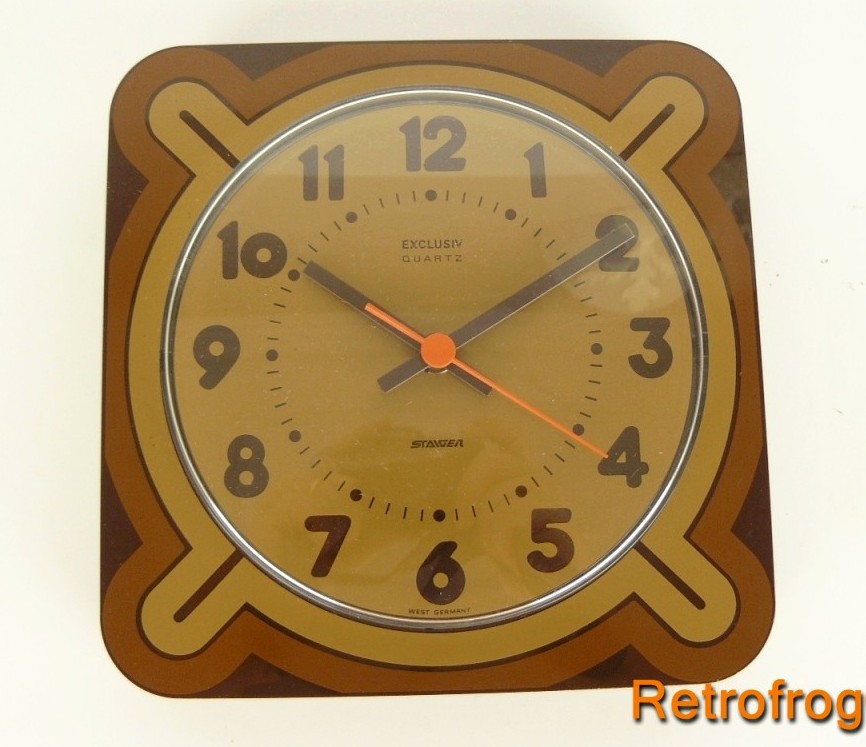This is an image featuring a vintage-style alarm clock with a rich, tan-brown clock face. The clock is encased in a circular, silver-toned metal rim, giving it a timeless appearance. Dark brown numbers are prominently displayed on the face, with two black hands and an additional orange hand indicating the time. The clock is wrapped in both a brown border and a slightly lighter tan border, accentuating its retro aesthetic. The entire clock is framed by a white square border, providing contrast and highlighting its shape. At the bottom of the image, there is an artistic stamp that reads "Orange Retro Frog," adding a whimsical touch to the photograph. The overall design and details evoke a sense of nostalgia, reminiscent of classic alarm clocks from the past.